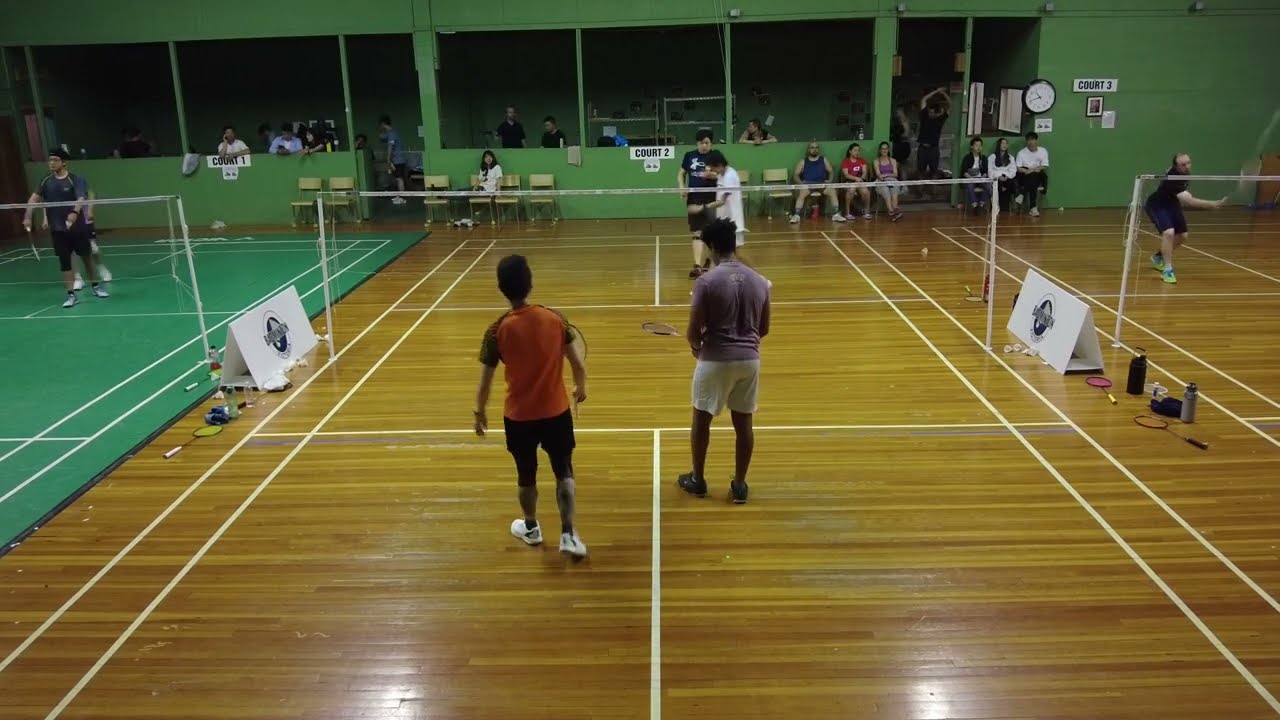This image showcases a bustling badminton tournament with three courts arranged in a row within a large gymnasium. The leftmost court features a green surface with white lines, possibly a tarp over the wooden floor, contrasting with the two courts on the right, which have brown hardwood floors marked with white badminton lines. 

In the center court, a doubles match is occurring. The players include two Asian boys in the foreground and two Asian individuals in the background, all dressed in shorts and t-shirts of various colors: orange, black, purple, and white. The far team appears to be preparing to serve while the near team readies to receive. On the leftmost green court, another doubles match is visible, while on the rightmost court, a single player, a large man in a black t-shirt and matching shorts, is making a shot.

The backdrop features a distinctive green wall that not only houses signs for courts 1, 2, and 3 but also includes cutouts serving as viewing areas. These areas seem to accommodate press members, coaches, or spectators who are positioned behind the players. In front of the wall, there are additional seating arrangements where people are engaged in watching the games. To the right of the image, a clock is visible, adding to the organized feel of the tournament. The gymnasium, though active with participants and onlookers, does not appear overly crowded.